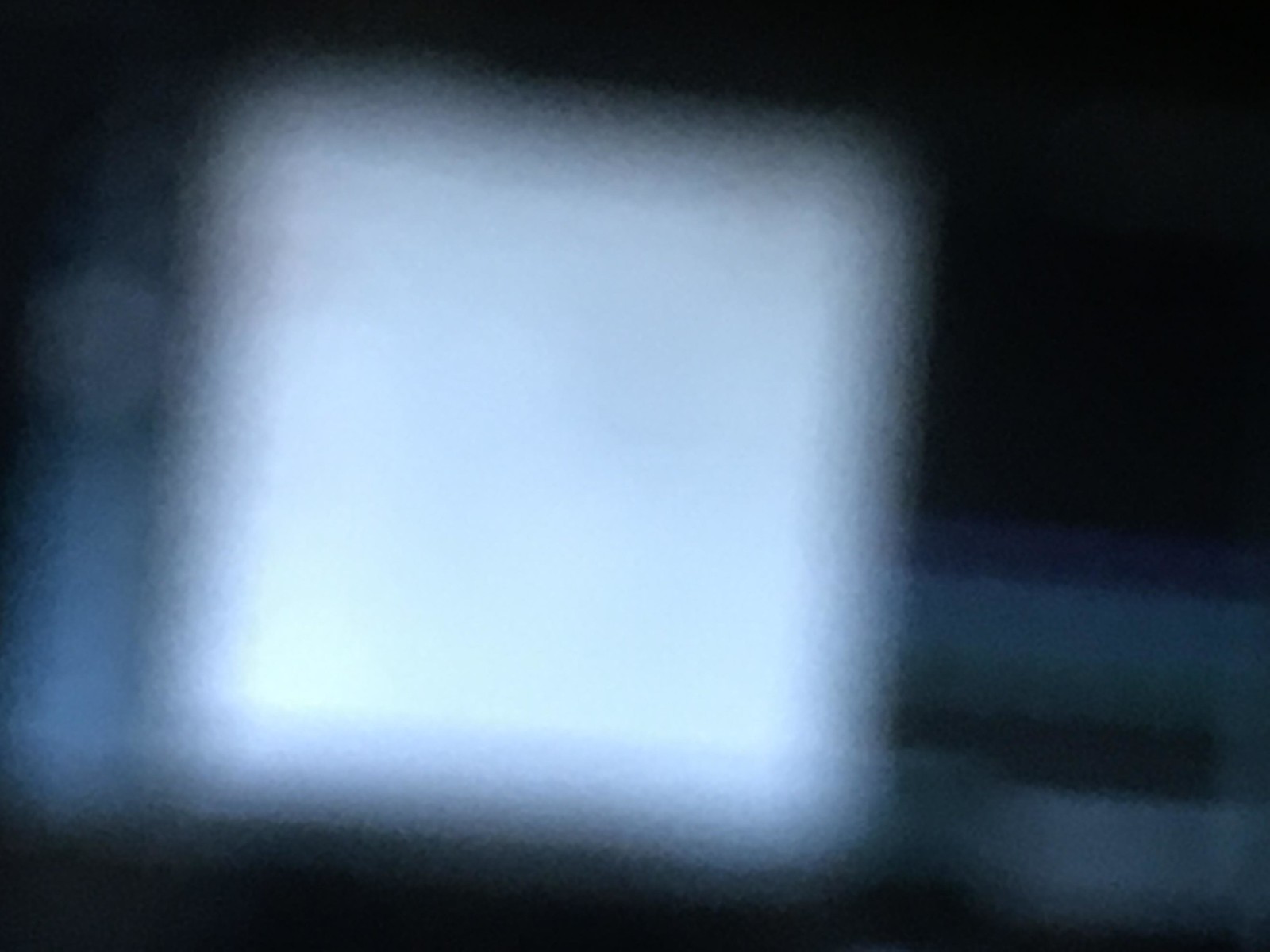The image is a very blurry, digital color photograph taken at night, possibly outdoors. Dominating the center is a slightly off-center, perfectly square object that resembles either a computer monitor or a TV screen. This square emits a white, fuzzy, and slightly grainy glow, with the brightness transitioning from white to light yellow towards the center. The background is a stark, flat black, suggesting it was taken in a dark setting with no natural light. 

In the bottom left corner and behind the left edge of the square, there is a noticeable blue blur, adding a slight color contrast to the predominantly dark and monochromatic theme of the image. Despite the heavy grain and blur, there’s a shadowy outline around the square, contributing to an overall artistic feel. No distinct details or subjects such as people are visible, strengthening the impression that this photograph captures the illuminated object in an otherwise pitch-black environment. The blurred and streaked lights enhance the abstract, almost surreal quality of the image.